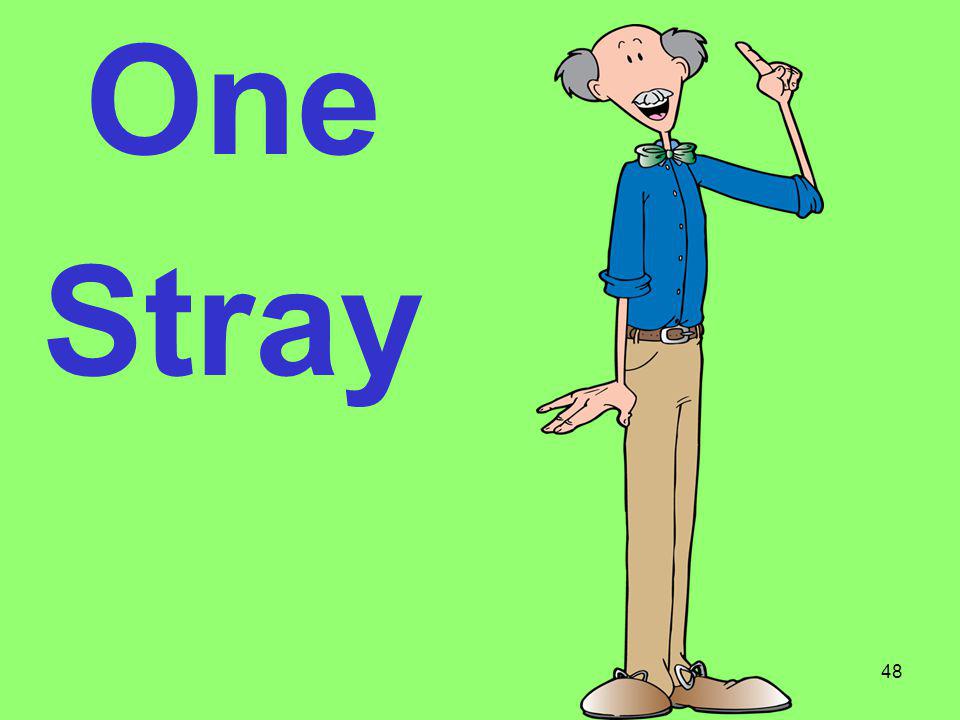The image features a cartoonish drawing of an elderly, slender man, wearing khaki pants with a brown belt, brown shoes, a blue button-down shirt with his sleeves rolled up, and a green bow tie. He has male pattern baldness with hair on the sides of his head, a thick white mustache, tiny dot-like eyes with thin eyebrows, and his mouth is open in a smile as he holds one finger up, as if making a point. The background is a bright neon lime green, with dark blue text in the upper left corner that reads "one stray," and a small number "48" in the bottom right corner. This image appears to be part of a magazine or book page.